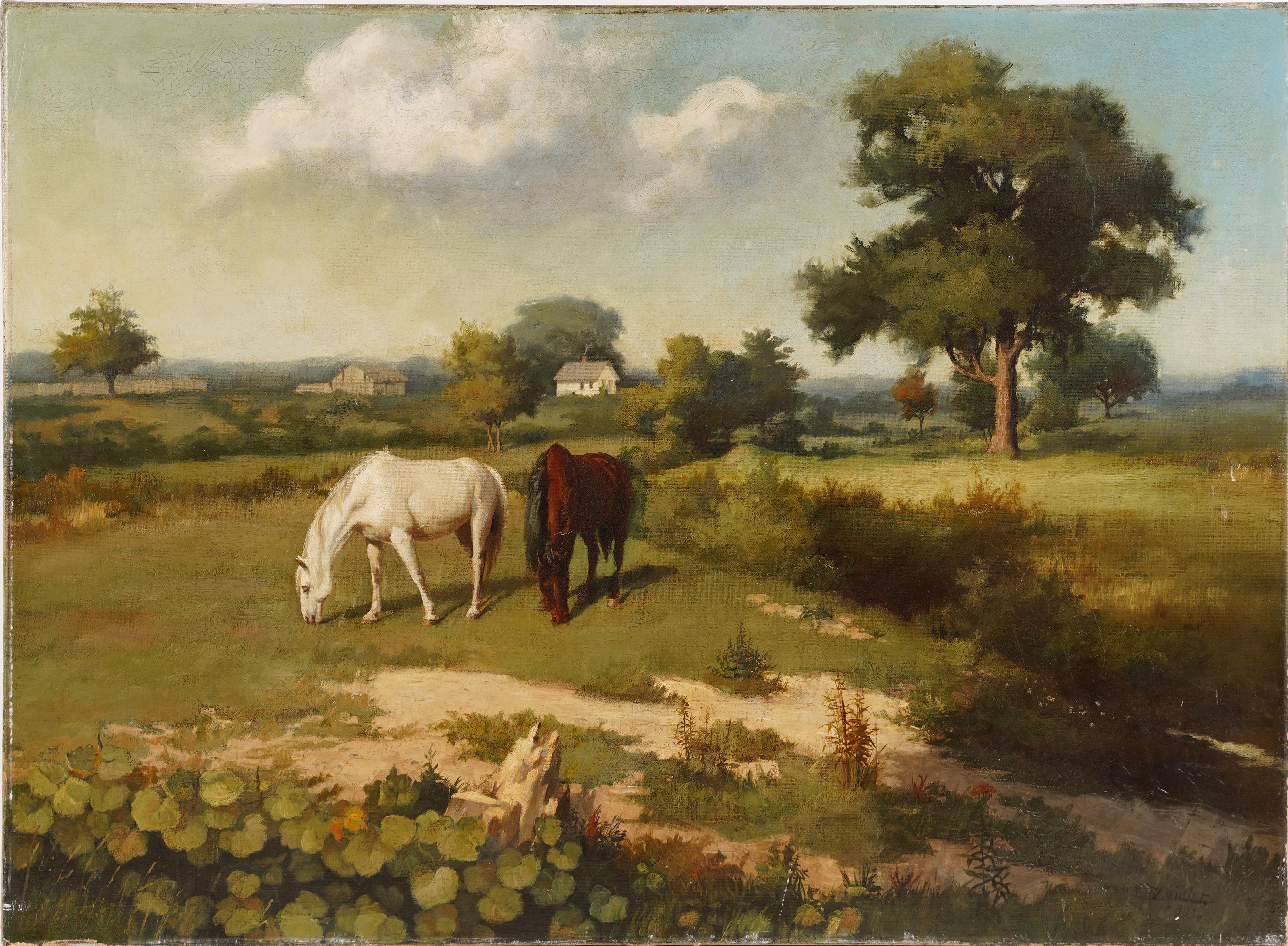The image depicts a beautifully detailed oil painting, possibly turned into a postcard or print, illustrating a serene meadow scene in early fall. At the center of the painting, two horses are prominently featured, both grazing quietly. The horse on the left is white, while the one on the right is dark brown with a black mane and tail. They are surrounded by lush greenery, including expansive fields of grass and scattered rows of bushes. Tall trees dot the landscape, adding to the sense of peacefulness.

In the background, there are a few farmhouses or homes: a small white house with a gray roof and a larger gray barn-like structure. Further in the distance, subtle rolling hills can be discerned. The sky is a gradient from light beige on the left to blue on the right, interspersed with puffy white clouds, enhancing the natural and bright ambiance of the scene. The overall clarity of the painting is remarkable, capturing the essence of a tranquil countryside with vivid color and detail.